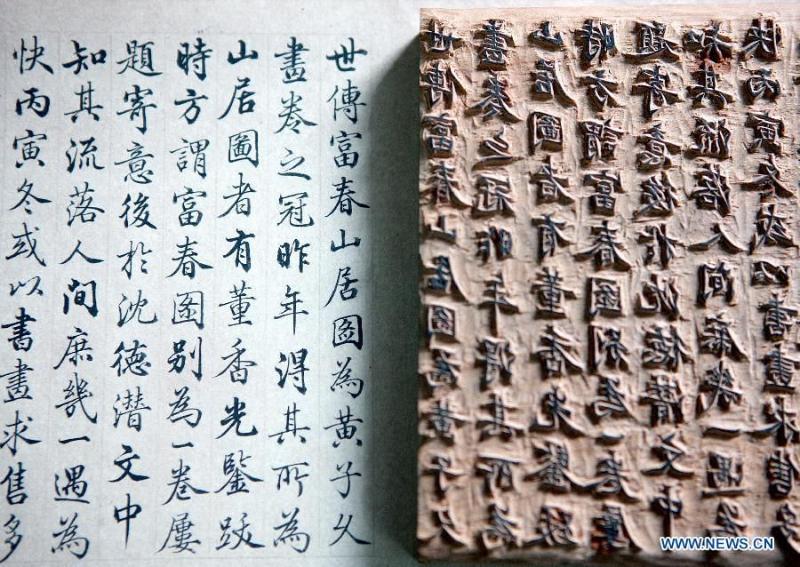This image features a detailed comparison between written and stamped Chinese characters. On the left, there's a white piece of paper with seven columns of Chinese text organized within grid lines, written in blue against a light blue background. On the right side, there's a tan and brown rubber stamp that has meticulously etched Chinese characters. The characters on the stamp appear to match those on the paper, suggesting that the stamp was used to create the printed text. Notably, the characters on the stamp are raised, having been carved out around them, rather than into the stone. In the bottom right corner of the image, the URL www.news.cn is prominently displayed in blue text with a white outline.